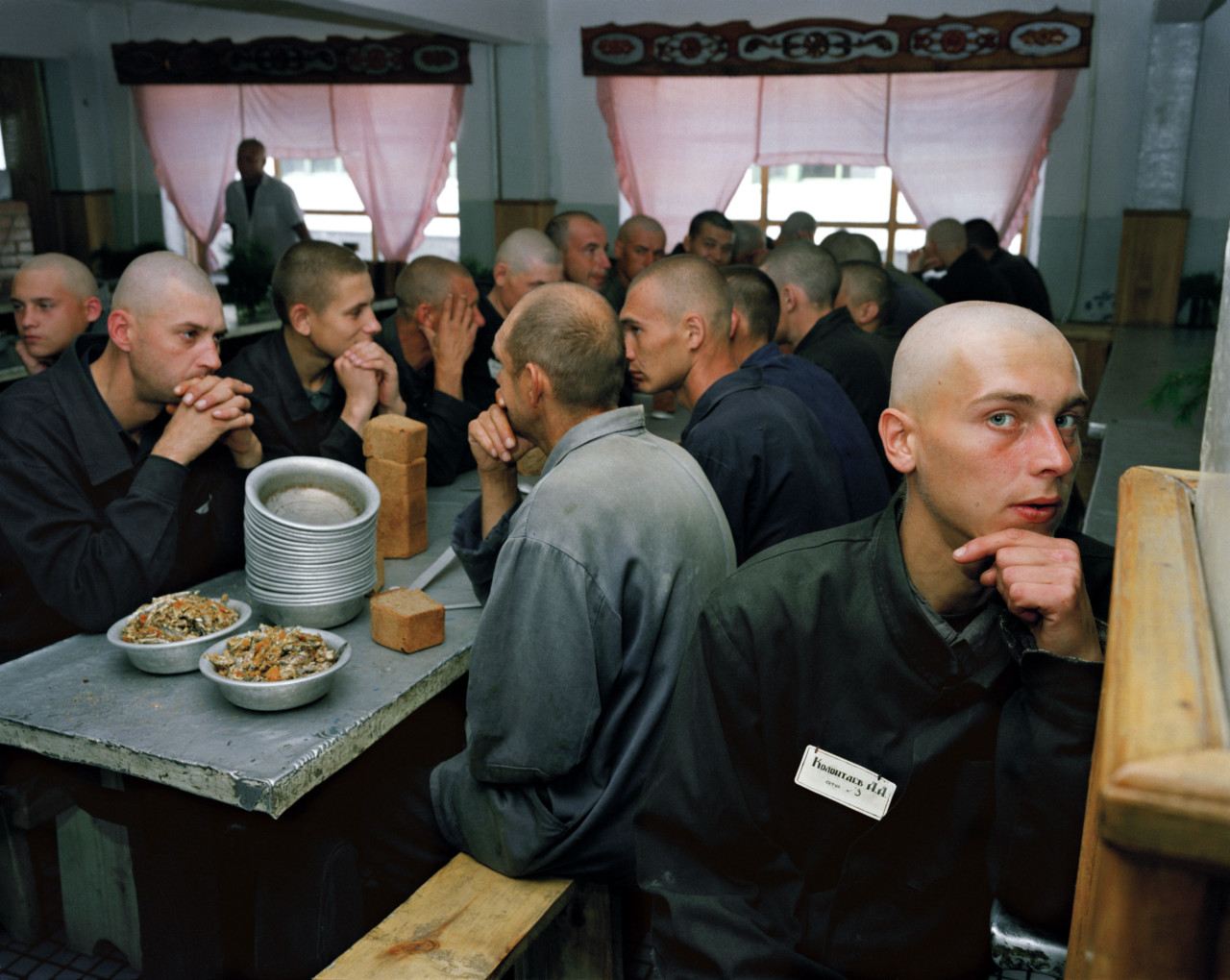The image depicts a group of white men, all with shaved heads or very short hair, seated inside a light gray or blue-gray room. This setting resembles a mess hall, possibly within a prison or a monastery. They are all dressed in long-sleeved jumpsuits, either in dark gray, dark blue, or black. The men are arranged around a gray, metal table with brown wooden benches, where several rusted metal bowls are stacked, and two bowls contain a colorful dish. Nearby, there are bricks of brownish bread. Most of the men are sitting with their hands folded in a manner that suggests waiting or praying. In the background, two windows with pastel pink curtains featuring ornate Asian designs adorn the room. Additionally, one man, who is not seated at the table, is looking at the camera, wearing a long shirt with a white badge.